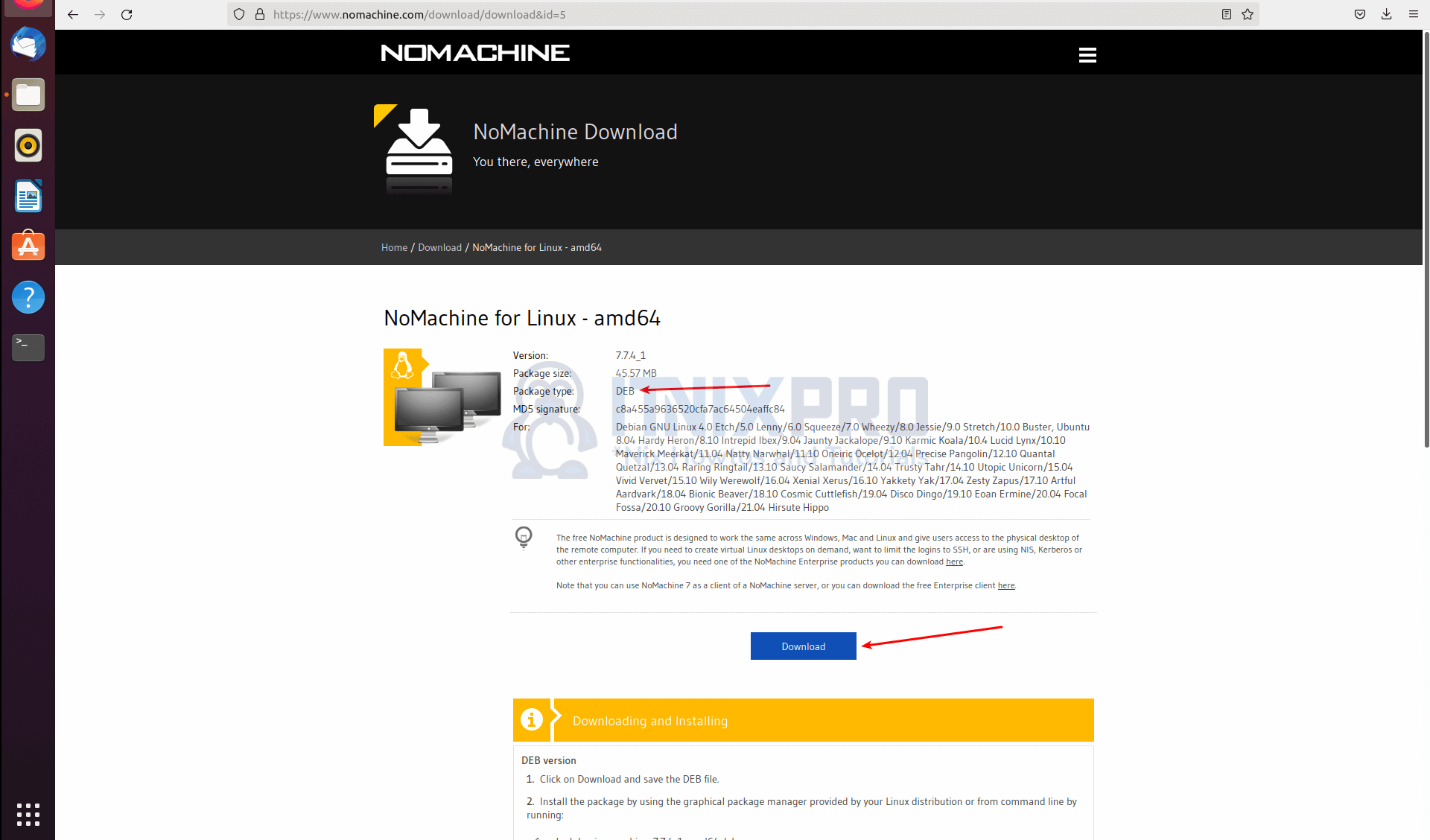This is a detailed screenshot of the NoMachine download page, specifically for the Linux AMD 64 version. The URL is www.nomachine.com/download/download?ID=5. In the upper left-hand corner, on a black header bar, there's the NoMachine logo featuring a white down arrow merged with a white computer icon. Next to the logo, the text "NoMachine Download" appears, accompanied by the tagline, "You there, everywhere."

The main content of the page indicates the following navigation path: Home > Download > NoMachine for Linux - AMD 64. The primary section of the webpage prominently displays the title "NoMachine for Linux - AMD 64." Below this, there's an image featuring two computers and the Linux Penguin mascot.

Further details include:
- Version: 7.7.4_1
- Package Size: 45.57 MB
- Package Type: DEB

A red arrow emphasizes the DEB package type, and another red arrow points to the blue "Download" button, guiding users toward initiating the download process.